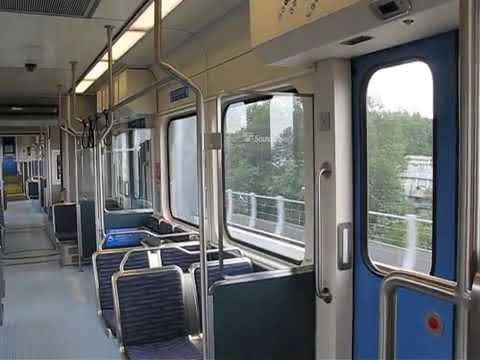The image depicts an empty commuter train car in motion, as evidenced by the slightly blurred guardrails visible outside the windows. The car's interior features a combination of blue and purple seats, each outlined with metallic, silver-grey edges, which complement the overall metallic aesthetic of the car. The floor is a light bluish hue, while the ceiling is white and fitted with a black dome, likely housing a security camera. To the right, a prominent blue door with a large window and a red push button is visible. Outside, viewers can see lush green trees, a grayish building on the right, and another building on the left adorned with white wording at the top, further surrounded by foliage. The train's predominately silver metallic finish, alongside numerous poles and railings, underscores its modern, utilitarian design.